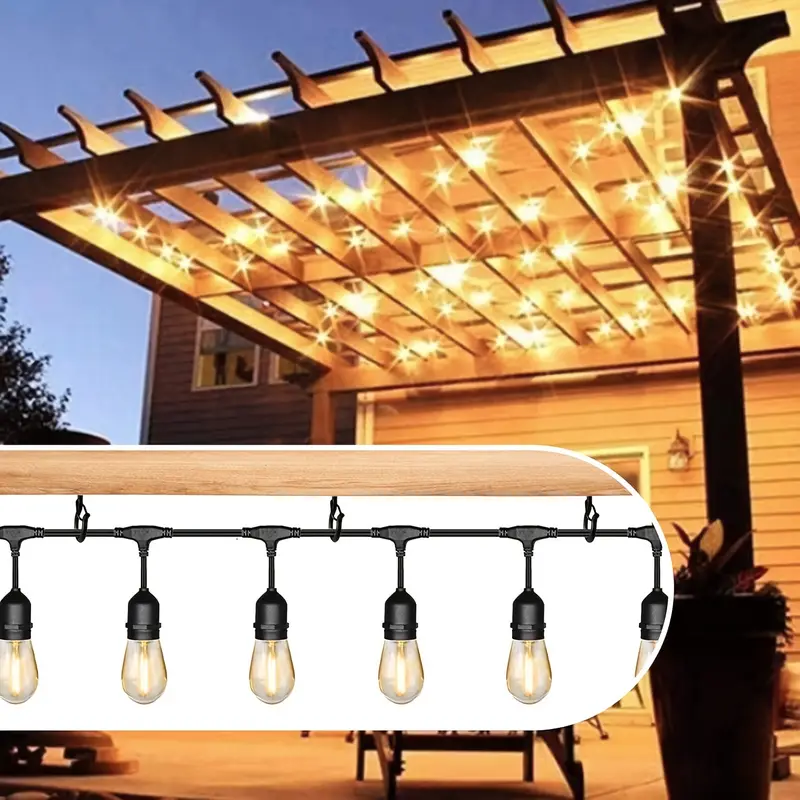The image depicts an outdoor patio area of a house, featuring a wooden arbor overhead that is densely adorned with bright, yellow incandescent light bulbs, casting radiant beams in all directions. The arbor's wooden rafters run horizontally and vertically, creating an open grid-like structure. The scene shows a mix of wooden and concrete textures, with wooden panels on the background wall—ranging from an orange hue to a darker brown color—and a concrete floor. On the left side, there's a tree and another section of the house is visible, while on the right, a tall potted plant stands near a supportive pillar.

Superimposed in the bottom left corner of the image is a prominent white section that spans from left to right and has a rounded edge. This section serves as a display area for light bulbs, featuring a light brown wooden bar at the top with three black hooks. Black wires hang from these hooks, each terminating in an outlet with a black wire leading to an incandescent light bulb. This overlay appears to be part of an advertisement, demonstrating how the light bulbs might be used in a real-world setting, echoing the illuminated arbor above.